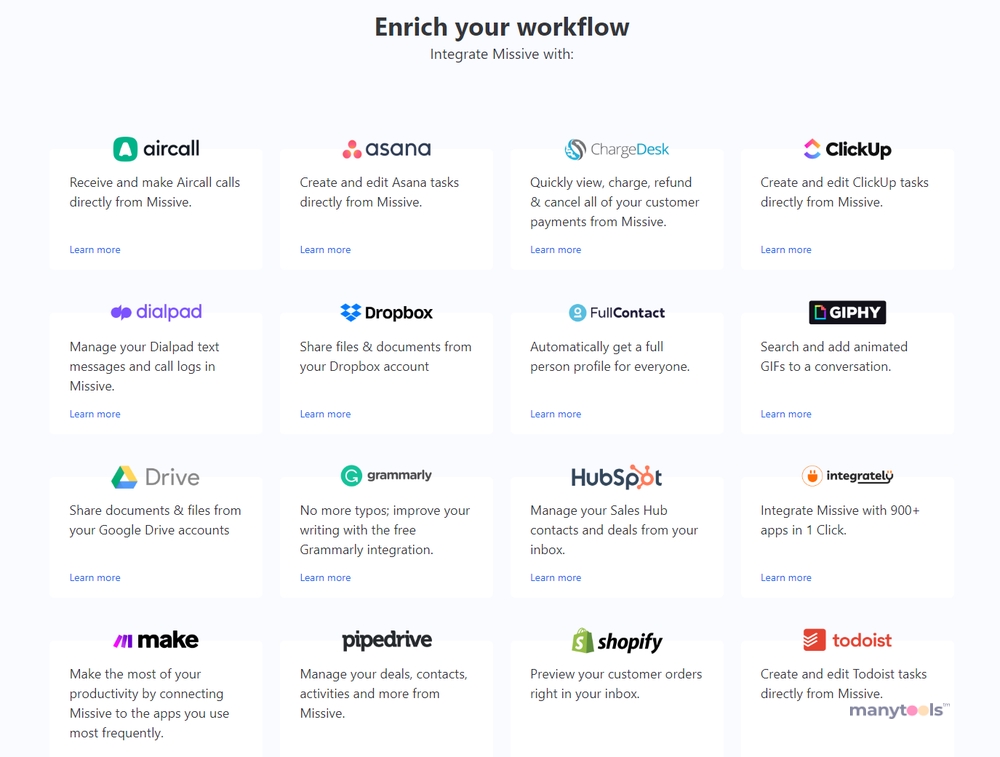This is a webpage from MISSIVE, featuring a pale, light blue background. Positioned centrally at the very top is a bold black text header that reads "Enrich Your Workflow". Directly below this, in slightly smaller black text, it says, "Enrich MISSIVE with:". The page showcases 16 individual white boxes arranged in a 4x4 grid. Each box contains the company name and icon at the top, accompanied by a brief description in light gray text about the integration benefits. 

From left to right, the integrations listed are:
1. Aircall
2. Asana
3. ChargeDesk
4. ClickUp
5. Dialpad
6. Dropbox
7. FullContact
8. GIPHY
9. Drive
10. Google Drive
11. Grammarly
12. HubSpot
13. Integrately
14. Pike
15. Pipedrive
16. Shopify
17. Todoist